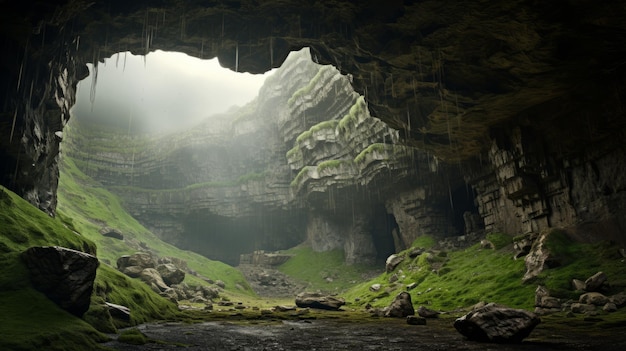This vivid, full-color photograph captures the mystical and rugged interior of a cave, bathed in natural daylight. The image, oriented horizontally, presents a detailed view of the scene both inside and outside the cave. The photograph reveals a substantial opening on the left side, through which light from an overcast sky streams in, illuminating the cave's lush green moss-covered rocks and patches of grass. The foreground is littered with loose stones, and there's an uneven, rocky surface from where the photo was taken. The lower portion has a mysterious, gray area suggesting either shadowed rock or possible water, untouched by sunlight. Stalactites hang from the cave ceiling, contributing to the magical atmosphere, while a slight mist gives the scene a foggy, ethereal quality. A steep, rocky hill leads up to the cave’s mouth, where the interplay of light and shadow highlights the layered rock formations. This image evokes a sense of deep enchantment and the natural beauty of the cave's hidden wonders.